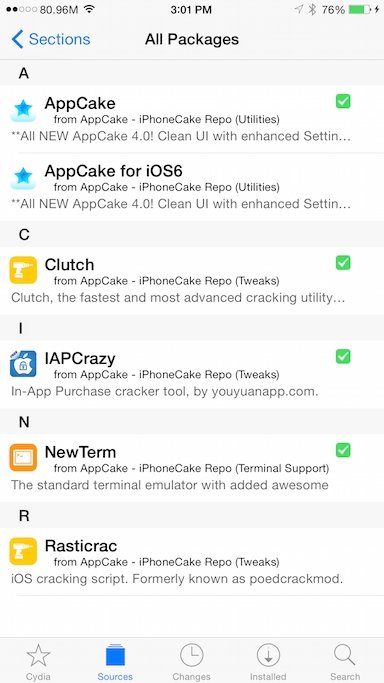Caption:

This is a detailed screenshot from a mobile device displaying the "All Packages" section of the AppCake application. The interface features an alphabetical listing of packages available within the app. Under the letter 'A,' users can find packages labeled "AppCake" and "AppCake for iOS 6." Moving to the letter 'C,' there is an option named "Clutch." Under 'N,' the package "New Term" is listed, and under 'R,' there's "Rastacrack." Additionally, the bottom navigation bar of the app includes functional buttons such as "Sources," "Changes," "Install," and "Search." These buttons provide users with various navigation and functional options within the app.